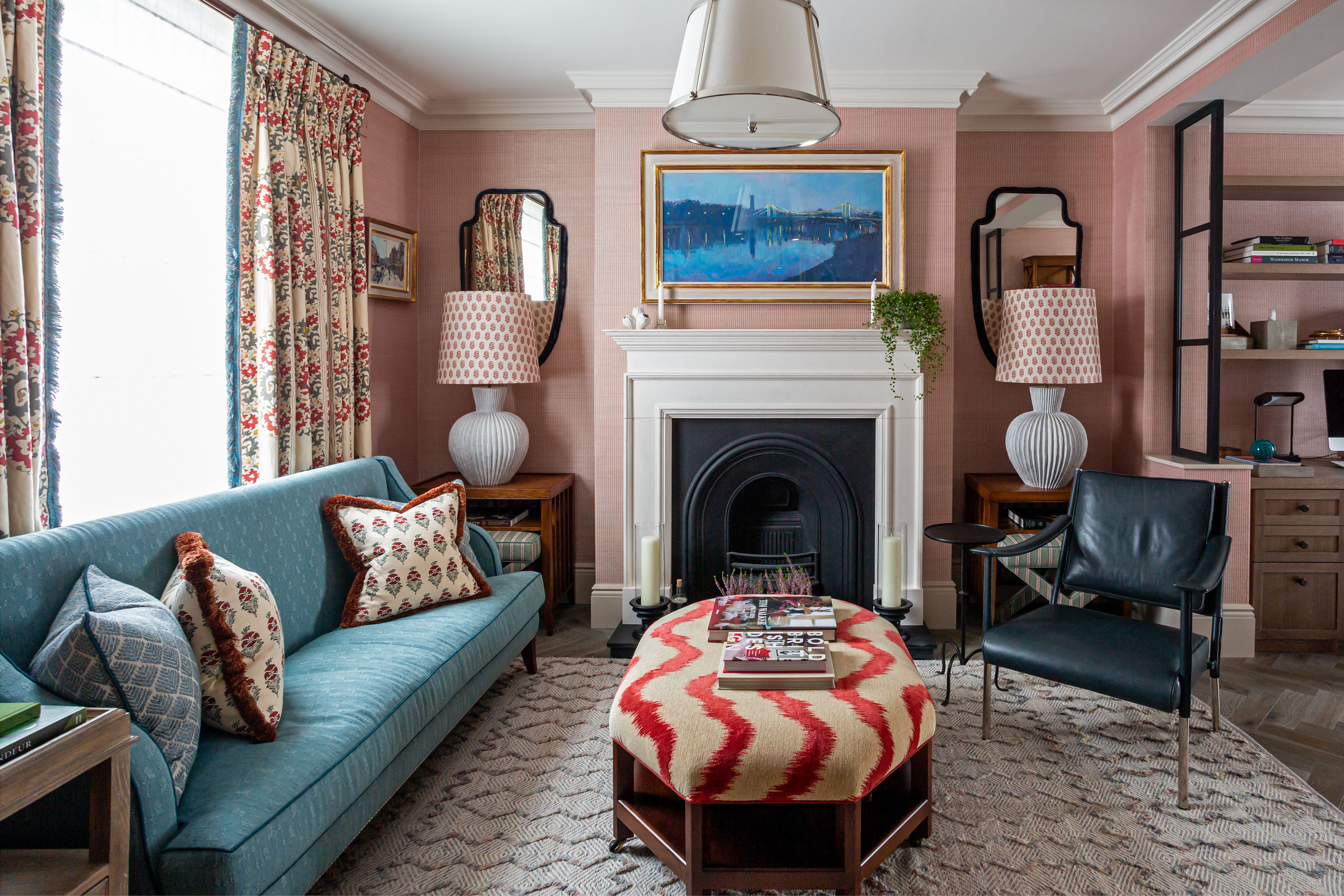This image depicts a detailed and ornate living room bathed in natural light coming from a heavily opened window draped with white curtains adorned with orange and blue floral patterns. In front of the window sits a large blue couch with three cushions: a plain blue one on the left and two identical ones with brown edges and central patterns. Dominating the center of the room is a long coffee table with a beige top featuring wavy line patterns, and behind it, a striking black fireplace with a white mantle.

Flanking the fireplace are two cream lampshades with faded orange polka dots. A lush green hanging plant and an unlit white candle sit on the right side of the mantle, while the left side features a white decoration and another white candle. Above the fireplace, a large rectangular painting of an ocean, beautifully framed with a gold-trimmed white frame, catches the eye. The fireplace itself has an arching black interior, and the surrounding wall is a soft pink hue, adding an additional layer of warmth.

The flooring is accentuated by a large white rug with a silver zigzag pattern. At the center lies a uniquely designed coffee table with a wooden base and a fabric seat featuring red wavy lines, on top of which rests a book. To the left side of the room, opposite the blue couch, is a thin, modern black leather chair with silver legs. On both sides of the fireplace are mirrors with arrow-like shapes enhancing the room’s symmetry and elegance. A hanging lamp in the middle of the ceiling completes the sophisticated ambiance of this lavish living space.